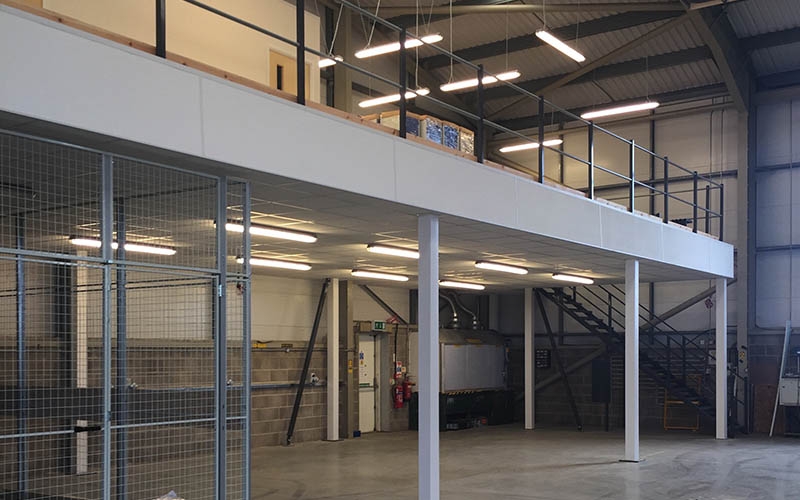This photograph depicts the inside of a warehouse, showcasing a detailed environment filled with various objects and colors. The central focus is a loft with a polished concrete floor, supported by white posts and enclosed by a metal railing. Above the loft is a yellow door on the wall, positioned in the top middle of the image. 

Descend to the middle and lower background areas where two fire extinguishers are mounted next to an emergency exit. The bottom portion of the wall is constructed from cinder blocks, forming a sturdy base. Metal steps are situated at the end of the loft, leading up to it from the background's right middle section. 

A chained fence can be seen, likely close to a metal cage on the bottom left, which is currently empty. The warehouse is illuminated by overhead lights, their positions scattered at the top of the image. The setting is painted with a palette of colors including gray, blue, red, orange, black, white, light yellow, and green, enhancing the industrial feel of the space.